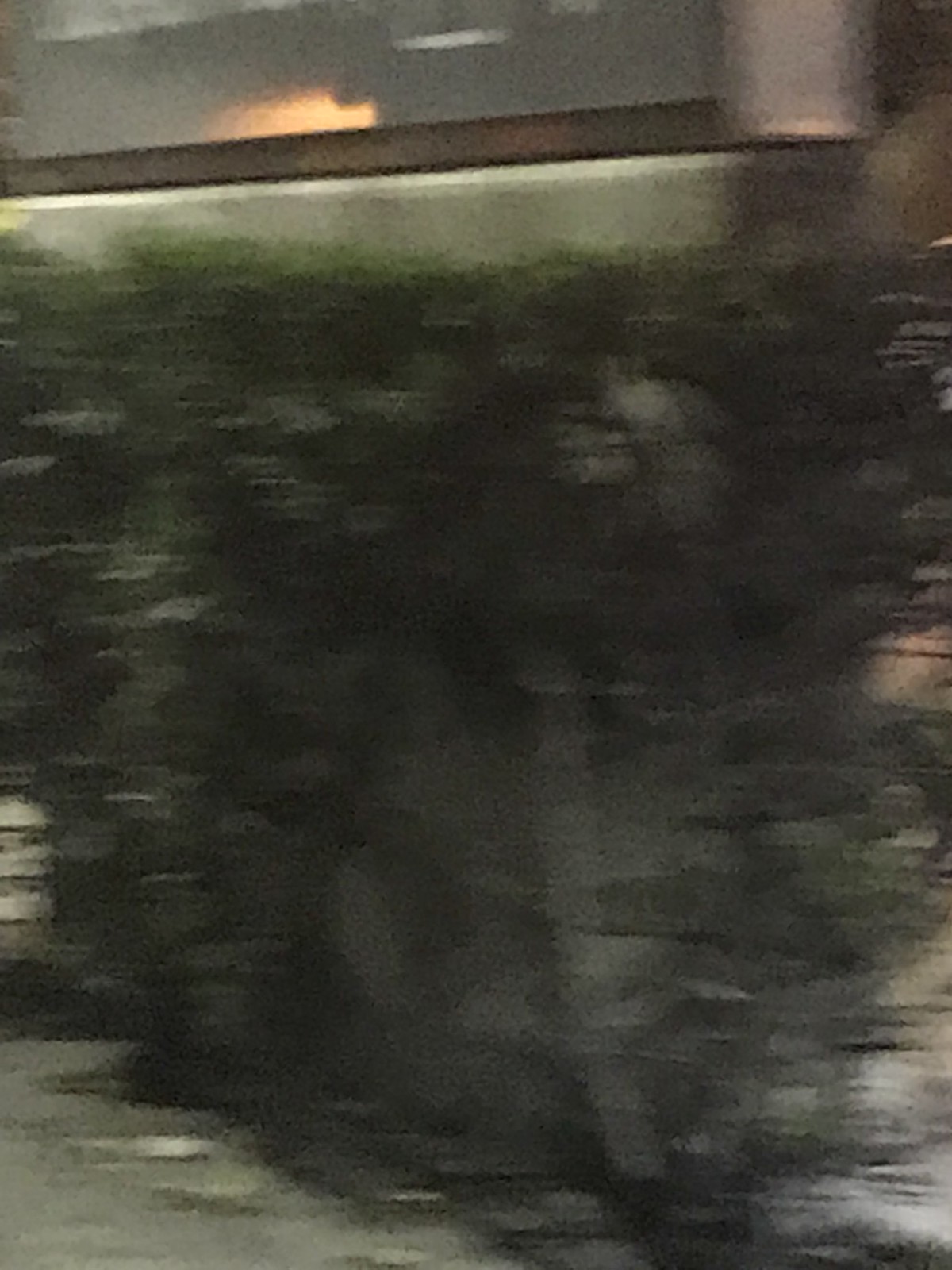In this nighttime photograph, a significant blur envelops the scene, shrouding its details and producing a dreamlike quality. Dominating the upper portion of the image, a grey block stretches horizontally from the left edge to the right, supporting a building perched on top. A strong light source illuminates the middle-bottom section of this building, casting an eerie glow against the surrounding darkness. Below the grey block, a row of blurry shrubs, likely evergreens, lines the base, adding a natural element to the urban landscape. In the lower left corner, a grey sidewalk is visible, scattered with some indistinct white objects. Above the sidewalk, protruding three white railings extend towards the left, adding linear interest amidst the otherwise indistinct and shadowy forms.